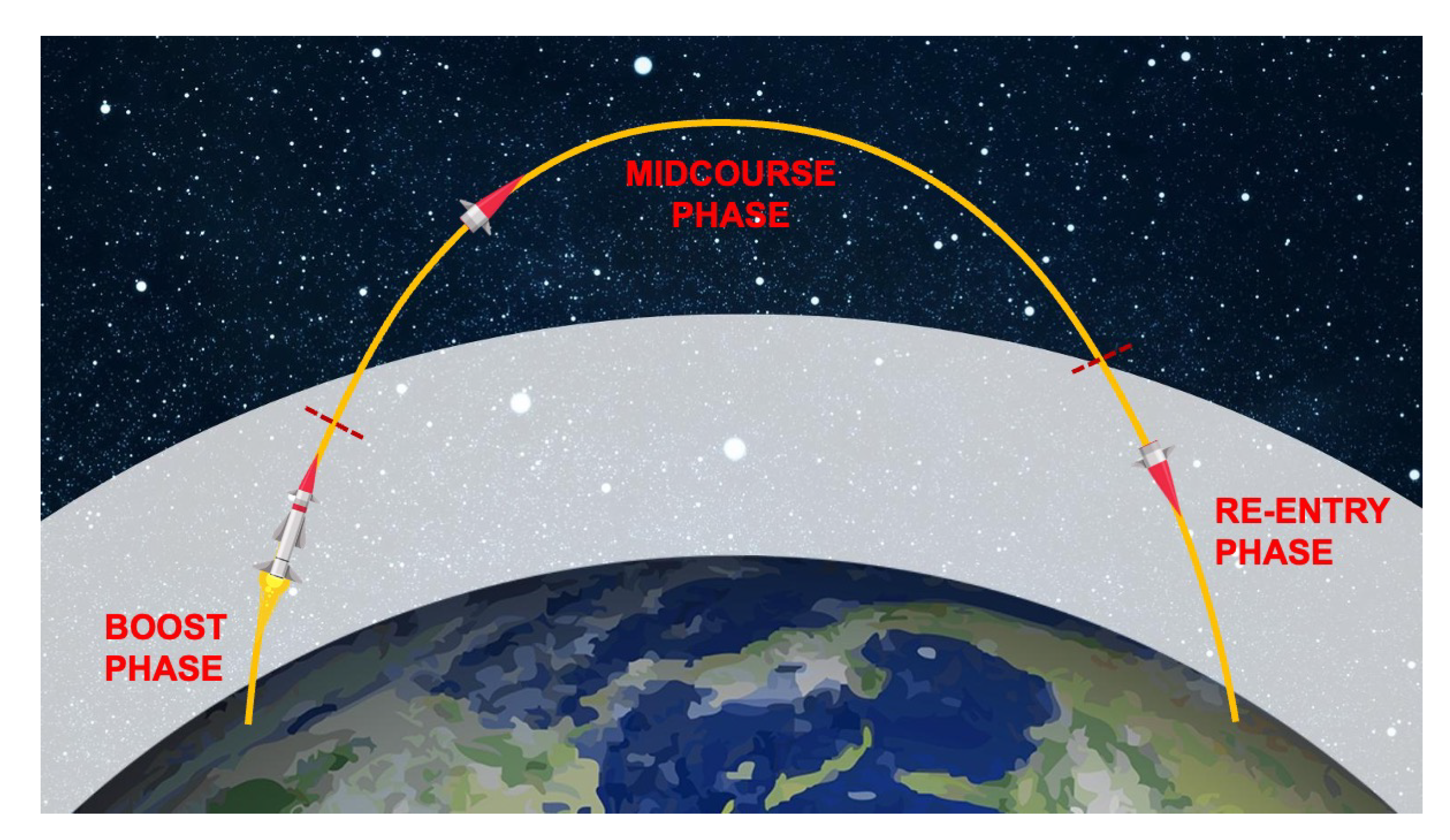The image is a detailed, computer-animated diagram illustrating the trajectory of a rocket. It is presented in a horizontal rectangular format. The top portion of the image is a dark blue, almost black representation of space, scattered with numerous white stars. Below this, a light gray arc spans from the bottom left corner to the upper right, partially transparent, allowing the stars to be seen through it.

Below this arc, the Earth is depicted with blue oceans and light green landmasses. On the left side of the Earth, slightly above the land, there is a white rocket with a red, triangular nose cone and yellow flames emitting from its rear. This initial section, labeled in red as the "boost phase," indicates the rocket's launch.

A prominent yellow arc outlines the rocket's path, arching upwards into space. As the rocket moves along this trajectory, the main body of the rocket detaches, leaving the red nose cone to continue along the path. At the peak of the yellow arc, the diagram marks this segment in red as the "mid-course phase."

The yellow arc then curves downward, ending back towards the Earth in the right section of the image. This final descent is labeled in red as the "re-entry phase." The image distinctly demonstrates each phase of the rocket's journey, from launch, through space, and finally returning to Earth.